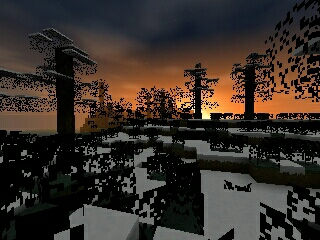The image, resembling a scene from a video game with rough, jagged graphics akin to Minecraft or a similar building game, is a horizontally oriented rectangle. Set outdoors within the game's pixelated world, the vibrant sky transitions dramatically from dark blue at the top to a reddish-orange gradient surrounding a bright yellow sun on the horizon, indicating either a sunrise or sunset. The upper portion of the sky also features scattered white clouds. In the background lie brown mountain ranges, adding depth to the landscape. In the mid-ground, a few black poles, each with small, grayish platforms, punctuate the skyline, with what appears to be black fragments falling from these elevated surfaces. In the foreground, the terrain consists of white, boxy foothills upon which the game's character stands, interspersed with green rectangular shapes that represent bushes. Trees constructed of stacked brown squares for trunks and green squares for leaves dot the landscape, contributing to the overall boxy and monochromatic appearance.